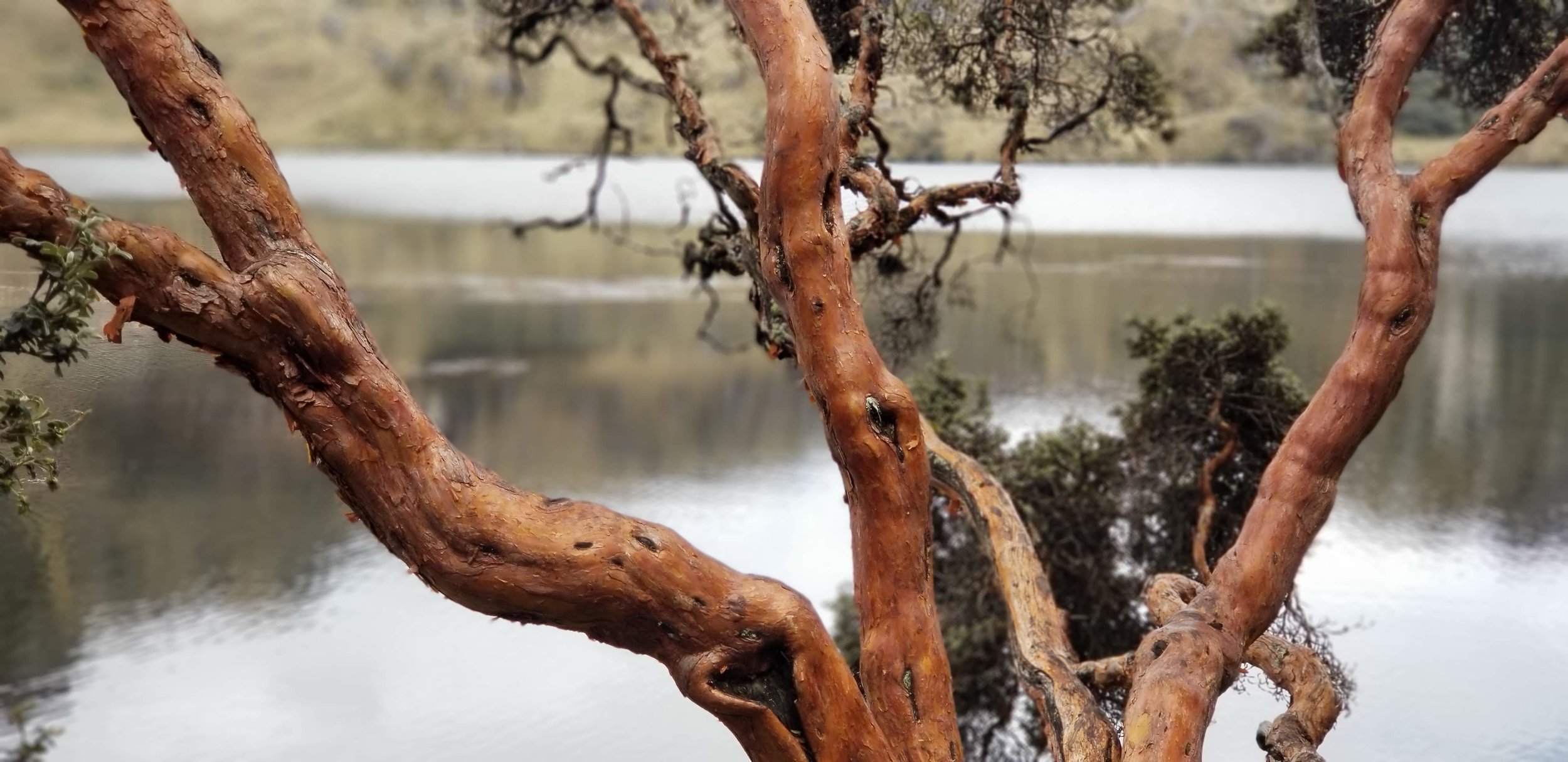This detailed nature photograph captures a tranquil scene by a large body of water, either a lake or a substantial pond. Dominating the foreground is a visually striking, not terribly tall tree marked by numerous large, prominent knots running up its textured, dark tan to brown trunk. From the main trunk, several curvy branches extend, numbering at least four, adorned sporadically with green leaves. These branches shoot out in various directions, allowing glimpses of the calm, grayish water in the background, which reflects the land on the opposite side. The distant shore appears to be a combination of brown grass and bushes, tinted with darker shades. The stillness of the water and the complete lack of wind contribute to the overall serene and undisturbed ambiance of the scene.